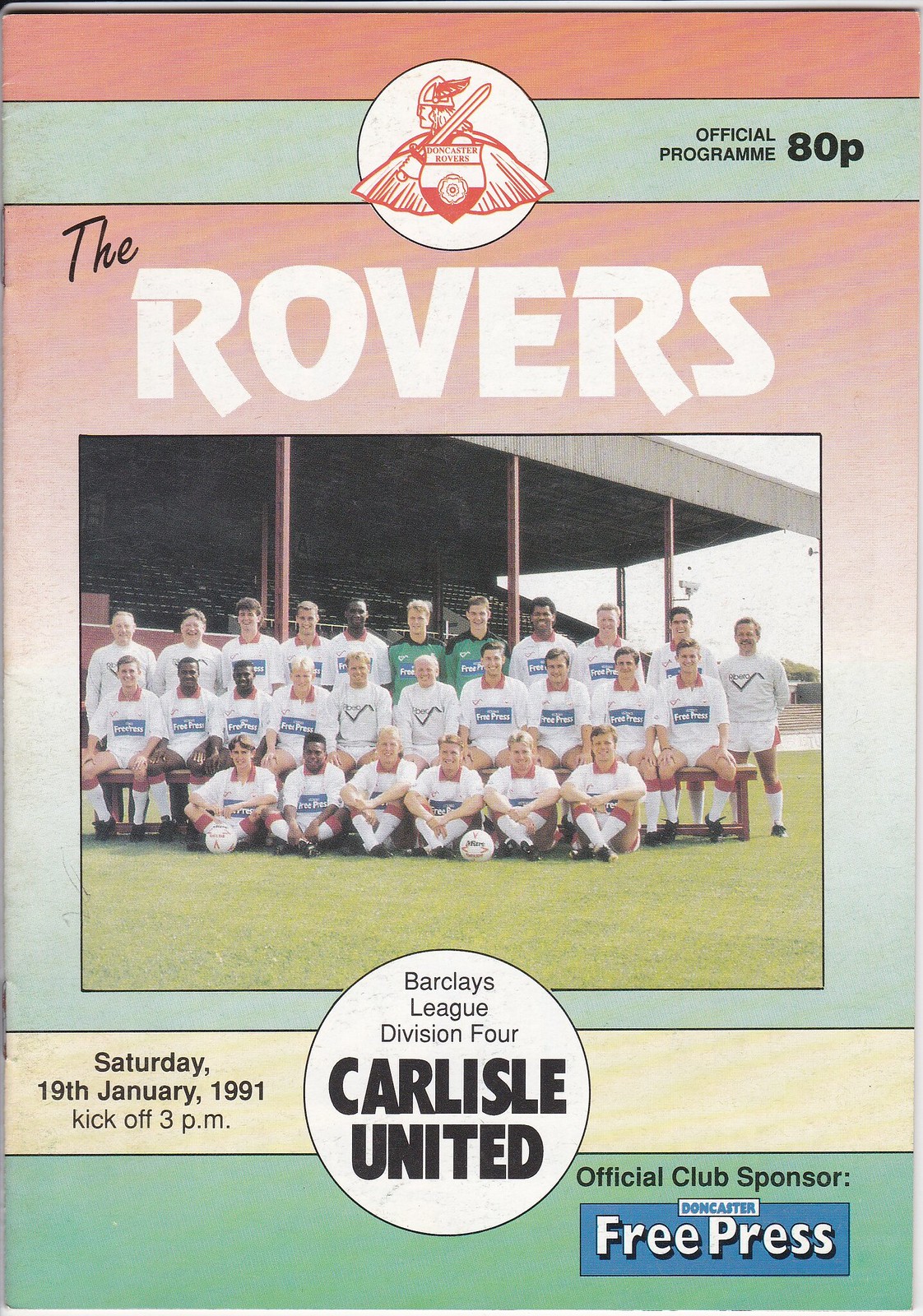This image is a scan of the front cover of a match day program for the Doncaster Rovers soccer team. The cover features a predominantly red and pink background with accents of green at the bottom. At the top, there's a detailed logo of a Viking warrior in red, wearing a helmet and a cape, holding a sword and a shield. Below the logo, the text reads "The Rovers Official Program ADP" in a distinctive style, with "The" in black and "Rovers" in white.

Central to the cover is a photograph of the entire team posing together. The players are wearing white outfits, while the goalkeepers in the back are dressed in green jerseys. They are positioned in front of a stadium with empty stands, suggesting it was taken on a sunny day due to the visible shadows on the field.

At the bottom of the cover, information about the match is provided: "Barclays League Division 4, Carlisle United, Saturday 19th January 1991, Kick-off 3 p.m." Additionally, in the bottom right corner, it notes the official club sponsor: "Doncaster Free Press."